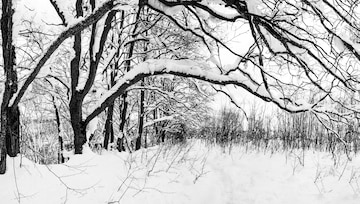This black-and-white photograph captures a serene, desolate winter scene. The image is wide and depicts an outdoor setting blanketed with heavy snowfall. Snow clings to the bare tree trunks and long branches that stretch from the left side of the image towards the top, cascading back down towards the right. More branches and brush poke through the snow across the landscape. The ground is thoroughly snow-covered, with scattered twigs and bare brush emerging intermittently. The sky is overcast and white, which creates a hazy gray tint over the entire scene, enhancing the cold, isolated atmosphere. In the background, distant trees or tall brush are faintly visible, adding depth to this stark, tranquil winter setting.